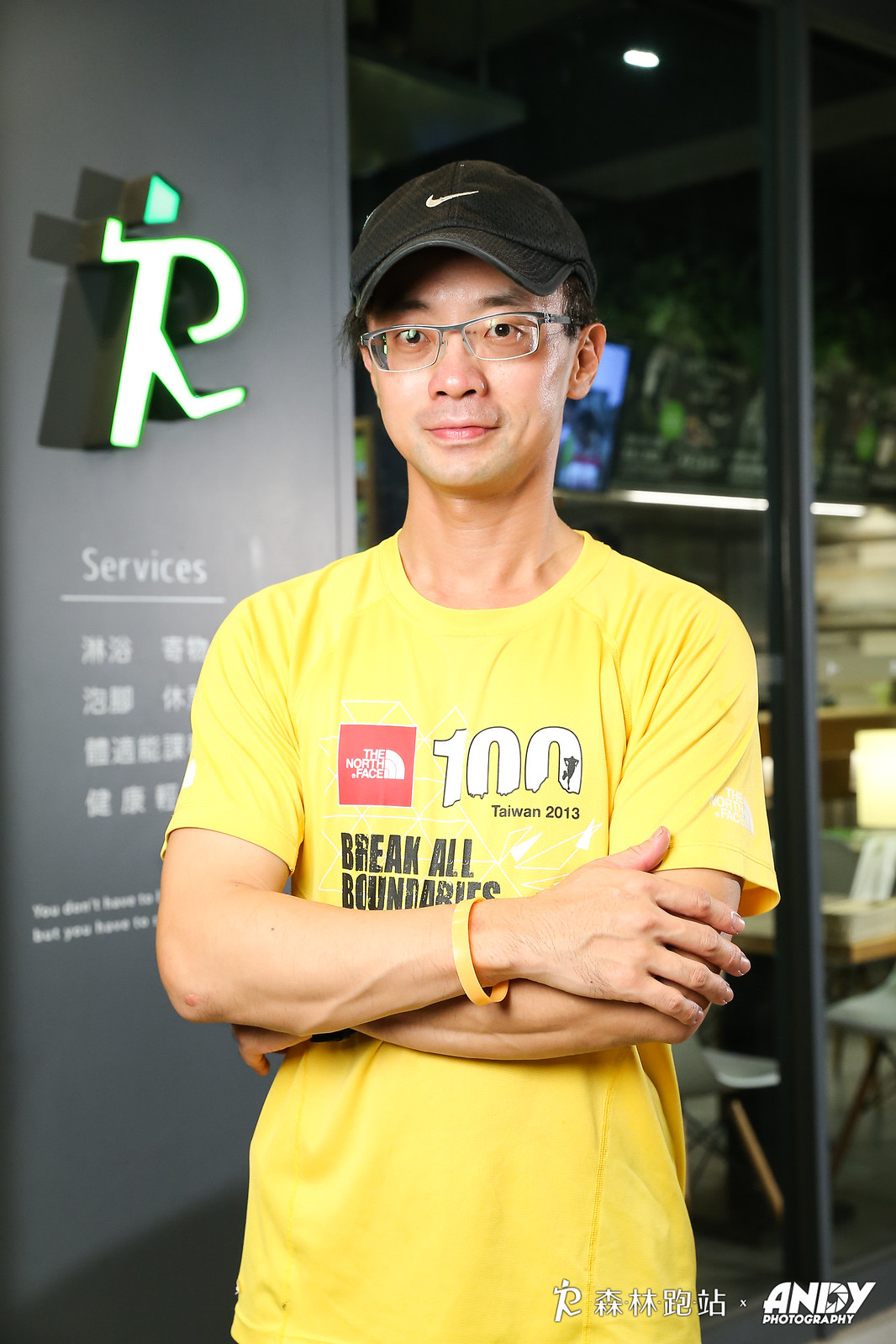The photograph is a high-quality, professional portrait of an Asian man standing with his arms folded. He is wearing a black low-bill Nike hat with a white checkmark and rectangular eyeglasses. The man is dressed in a yellow competition shirt, provided by The North Face, which prominently features the text "100 Taiwan 2013 Breaking All Boundaries." He also has a yellow rubber charity bracelet on his right wrist that matches his shirt. In the background, there is a light shaped like a running man accompanied by the word "services." Below this, a white and green 'R' logo is visible, part of a sign for a place that offers amenities like showering, storing luggage, foot massage, and entertainment. The setting appears to be a café or similar venue, with chairs and tables visible through a window. At the lower right-hand corner of the image, there is a watermark that reads "Andy Photography" along with some Chinese characters. The image dimensions are five inches wide by eight inches tall.